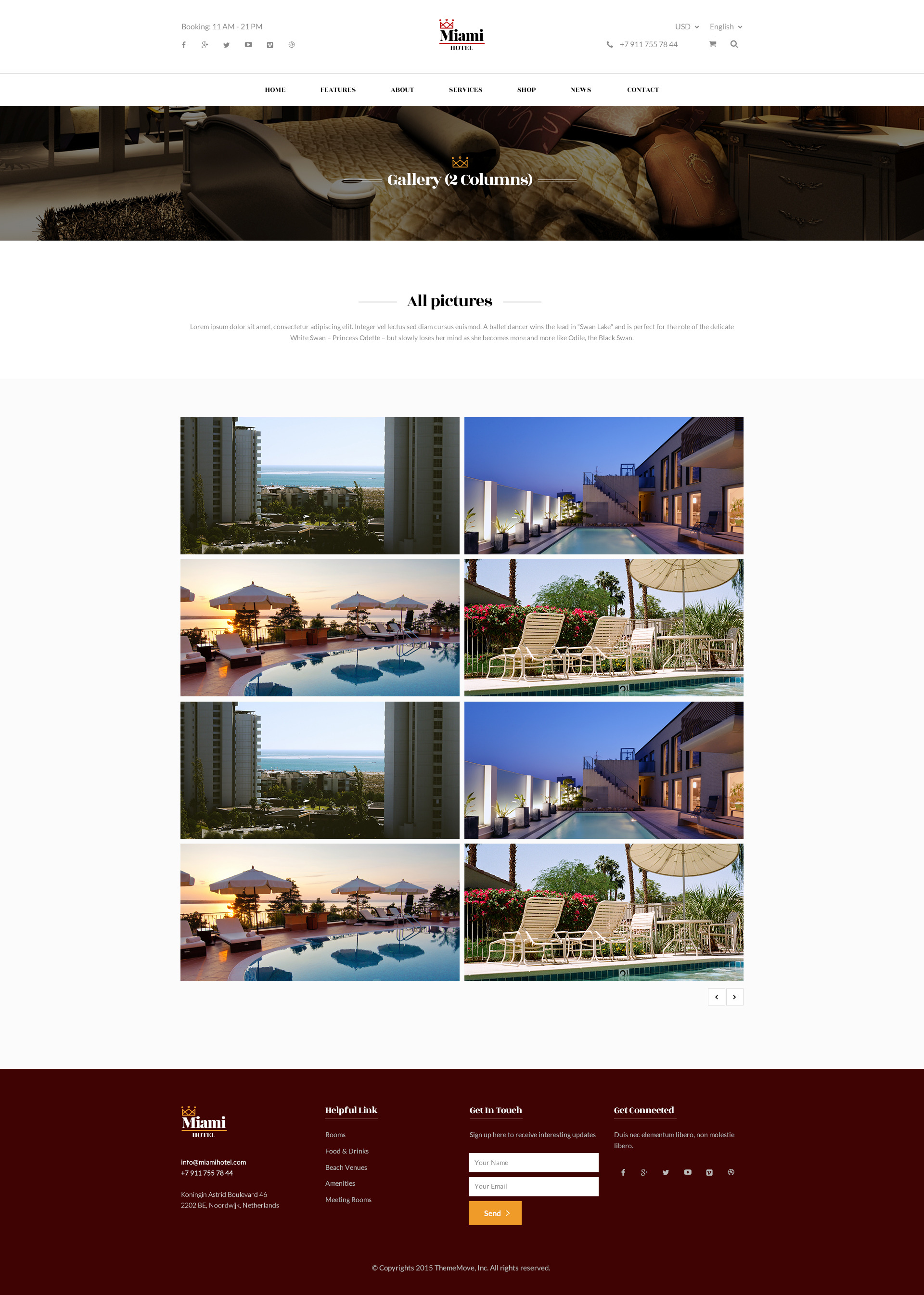The image is a screen capture of a web page from a Miami hotel. Centered at the top of the page, the word "Miami" is prominently displayed in black with a red crown perched atop the 'M', and the word is underlined with a red line. Directly below this, there is a banner featuring an image likely depicting a living room or bedroom area, furnished in beige, brown, and gold tones. Beneath this banner, the text "All Pictures" appears in black. Following this, eight images are arranged in two columns, with four images in each column. Upon closer inspection, the images repeat; the first and third rows display identical photos, as do the second and fourth rows. The pictures highlight a poolside scene and towering high-rise buildings.